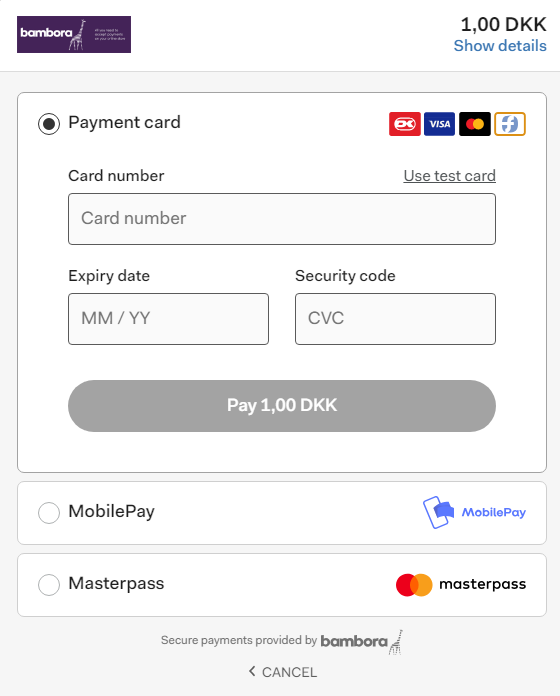A user is completing a purchase on an online payment platform. They have chosen to pay with a payment card from the available options—Payment Card, Mobile Pay, and Masterpass. The user is in the process of entering their card details, including the card number, expiry date, and security code. The amount to be paid is specified as 1,00 DKK, which is the currency of Denmark, with 1 DKK being approximately equal to 0.16 USD. The top part of the interface features a small logo of Bambora, a company known for secure payment processing, accompanied by an illustration of a giraffe. The text beside the image is too small to read clearly. At the bottom of the screen, there's a note indicating that the secure payments are provided by Bambora. The design of the payment interface is clean and minimalistic, with a primarily white background and light grey fields for input. The actual item being purchased by the user remains unspecified.